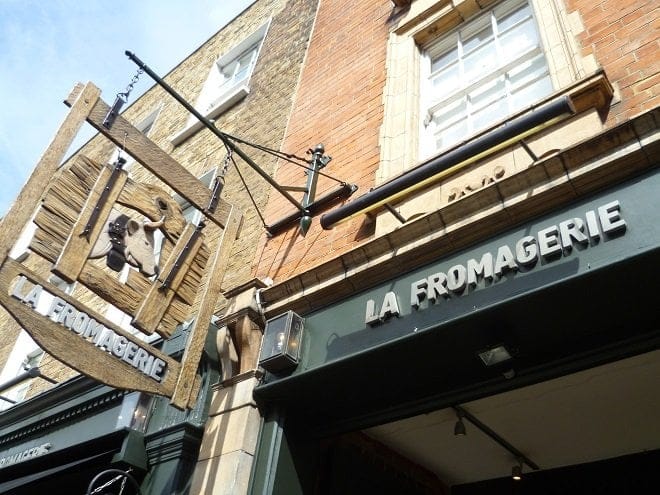This vivid color photo captures the upward-facing facade of a building set against a clear blue sky. The structure is a blend of red brick and beige stone, creating a rich, textured surface. Above the front doorway, a gray sign reads "La Fromagerie," while to its left, a gold metallic spoke protrudes from the building, supporting a wooden framed sign. This secondary sign features a sculpted side profile of a bull or cow, carved with the same text, "La Fromagerie." The scene includes a hint of a window, metal elements, and a light fixture on the left side. The overall look is cohesive, with tones of red, orange, and brown bricks, adding depth to the architectural details.